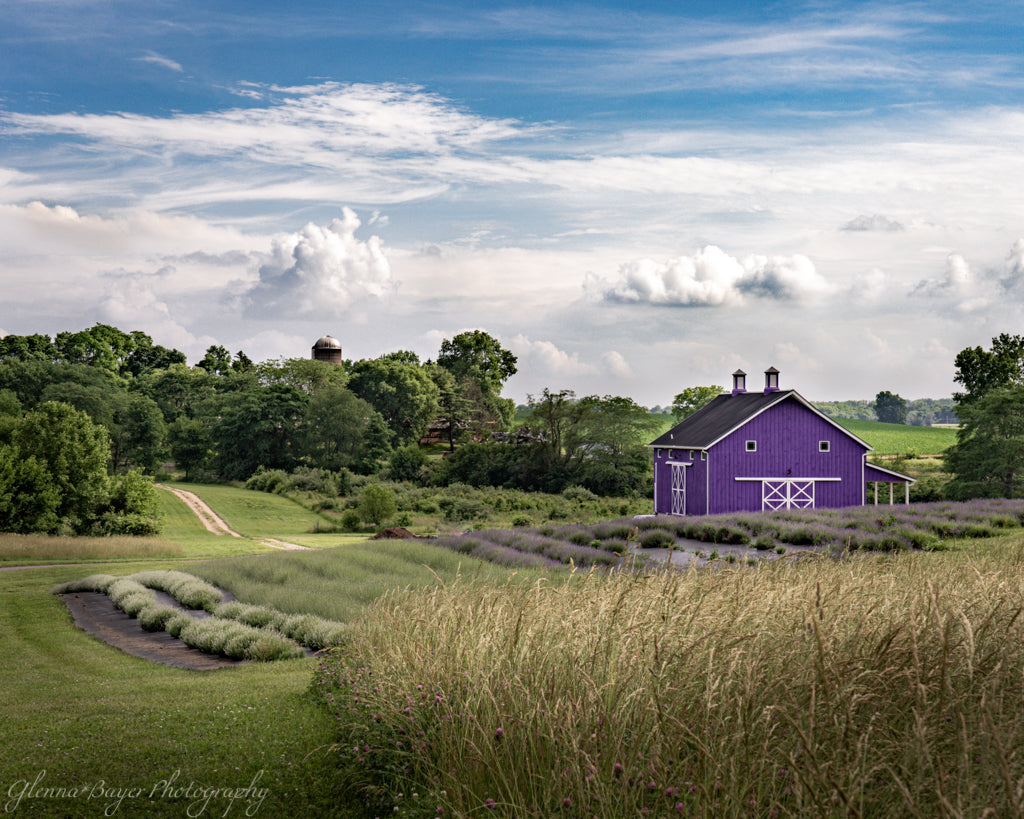The image depicts a pastoral countryside scene with a purple house, which features white-framed doors and small square windows above the entrance, located on the right side of the picture. The house has a striking black, triangular roof adorned with two chimneys. The surrounding farmland is lush with green plants and landscaped areas. In the foreground, rows of lavender bushes can be seen, although most are predominantly green with minimal lavender bloom. The lavender is bordered by tall grass or wheat fields, and a manicured lawn encircles the diverse vegetation. Toward the back of the scene, tall, vibrant green trees line the horizon, and the top of a grain silo can be glimpsed peeking above the foliage. The sky above is a mixture of blue and white, dotted with fluffy clouds. A subtle watermark reading "Glenabair Photography" is visible in the bottom left corner, hinting that this may either be a photograph, possibly enhanced by Photoshop or AI, or an artful painting.